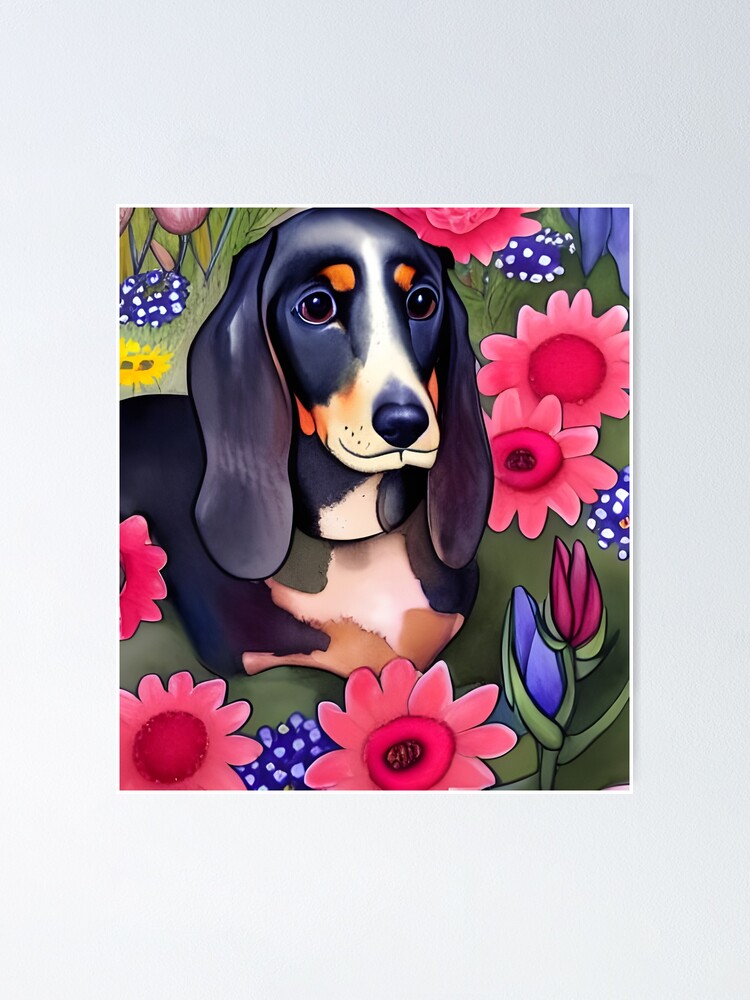This is a vibrant cartoon-style image featuring a dachshund-like dog prominently in the center against a large rectangular, grayish off-white background. The dog has a striking color palette: predominantly black with a lighter chest area that's a pinkish-beige, black face transitioning to a lighter off-white or yellowish muzzle, and brown eyes with brown eyebrows. It also has distinguishing brown spots above its eyes and very long ears. The dog is depicted laying down with its paws stretched out in front, surrounded by a vividly colored garden. The garden is lush with various flowers, including pink and blue blooms, as well as unopened buds of blue and purple irises. The pink flowers notably feature large centers, some with little black circles. The grass around the dog is green and closely cropped, creating a cleared, serene space that contrasts beautifully with the large, colorful flowers overlapping each other in shades of pink, blue, red, and purple, adding to the whimsical and detailed nature of the artwork.